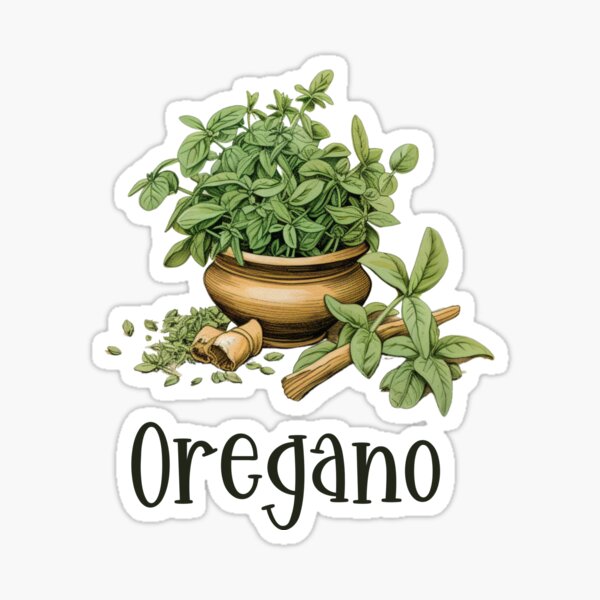The image depicts a detailed, hand-drawn decal or sticker of a vibrant oregano plant, housed in a brown, almost bronze-colored pot. The pot is intricately designed with lines that give it a subtle 3D effect. The lush green leaves of the oregano bush out from the pot, with additional leaves scattered around its base. Some leaves are chopped up and placed to the front and side of the pot. The illustration includes a trunk-like stem about the size of a finger, with smaller stems branching out and adorned with detailed leaves showing varied patterns. At the bottom of the image, the word "oregano" is inscribed in black letters, adding to the realistic yet cartoonish charm of the picture.